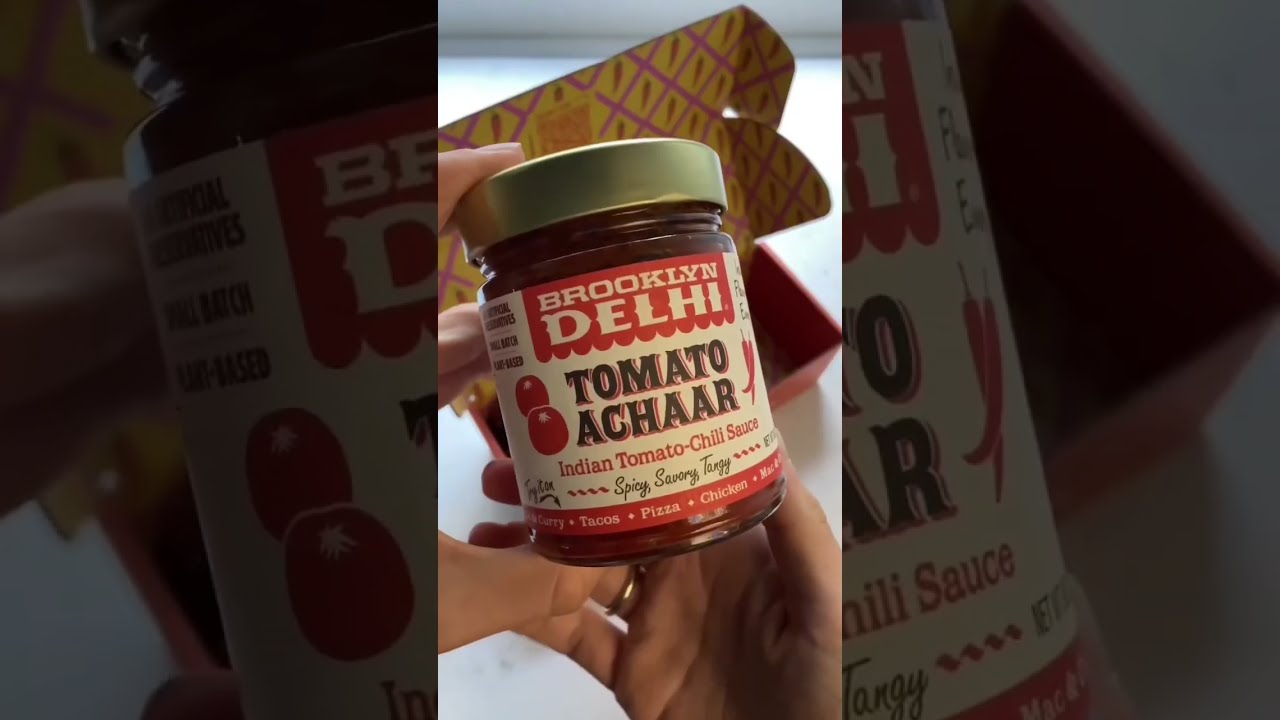In this close-up image, a person is holding a glass jar with both hands, prominently displaying a gold wedding ring on the ring finger of their right hand, suggesting the person is married. The jar, capped with a gold lid, contains a dark red sauce and features a predominantly white label with distinctive red and black text. The brand name "Brooklyn Delhi" is prominently displayed in bold, red letters within a white rectangle, and below it, the product title "Tomato Achar" is written in black with red highlights. This Indian tomato chili sauce is described as "spicy, savory, tangy." The label also includes illustrations of tomatoes on the left and chilies on the right, with usage suggestions such as tacos, pizza, and chicken highlighted at the bottom. In the background, there's a yellow packing box with pink stripes and pepper designs, indicating that the jar was recently unboxed.